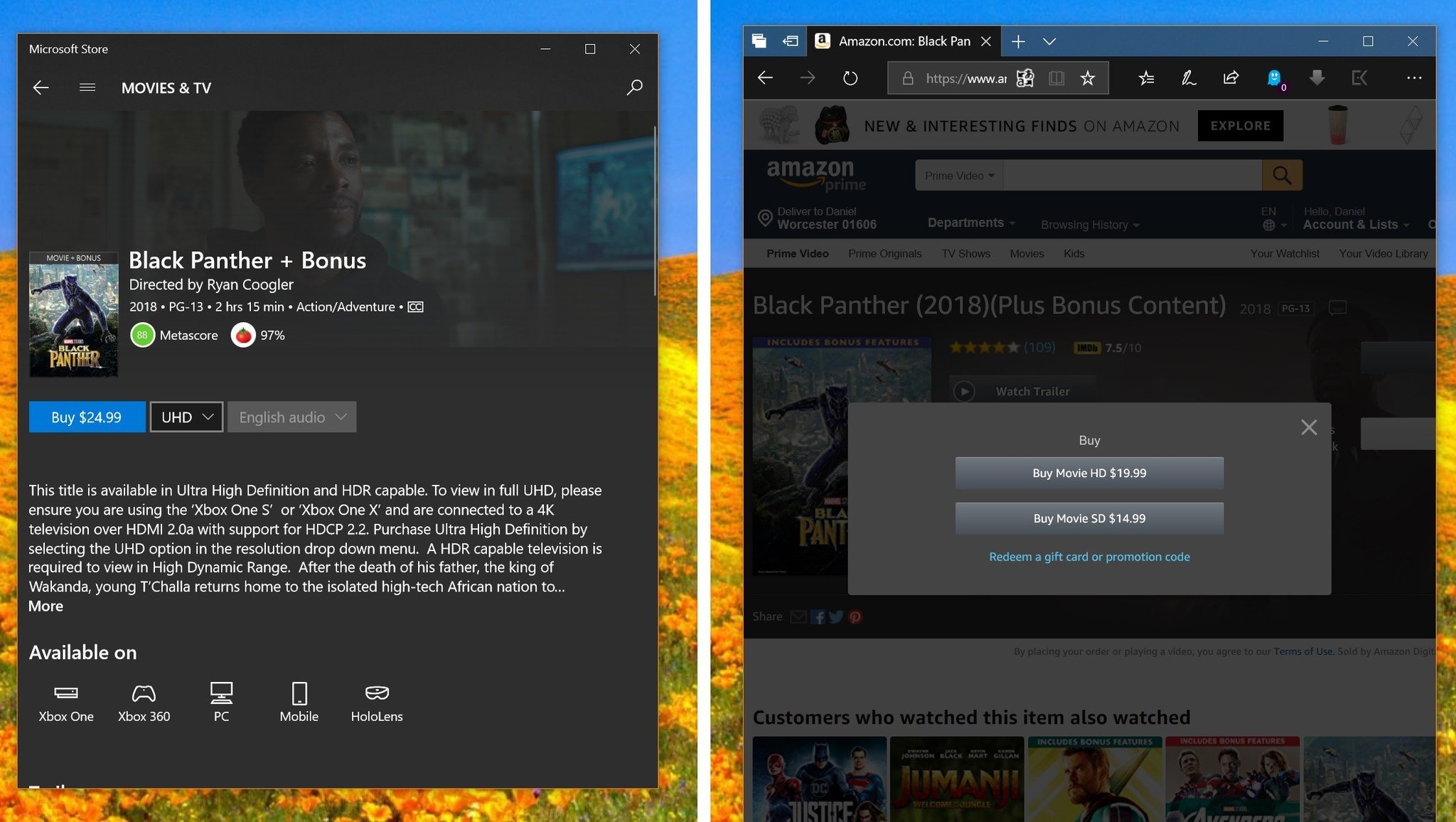The image features two boxes side by side. The left box showcases the movie "Black Panther" available on the Microsoft Store. It includes details such as the director (Ryan Coogler), release year (2018), rating (PG-13), duration (2 hours 15 minutes), and genre (Action/Adventure). The movie has an impressive Metascore of 97% on Rotten Tomatoes. The cover art of "Black Panther" is also displayed in this box.

Below the cover, there's a blue "Buy for $24.99" button. To the right of this button, there are drop-down menus: one labeled "UHD" and another for "English audio." The caption below these elements states that the title is available in Ultra High Definition (UHD) and HDR. It advises customers to ensure they are using an Xbox One S or Xbox One X connected to a 4K television with HDMI 2.0a that supports HDCP 2.2, to view the content in full UHD. To purchase the movie in UHD, users should select the UHD option from the resolution drop-down menu.